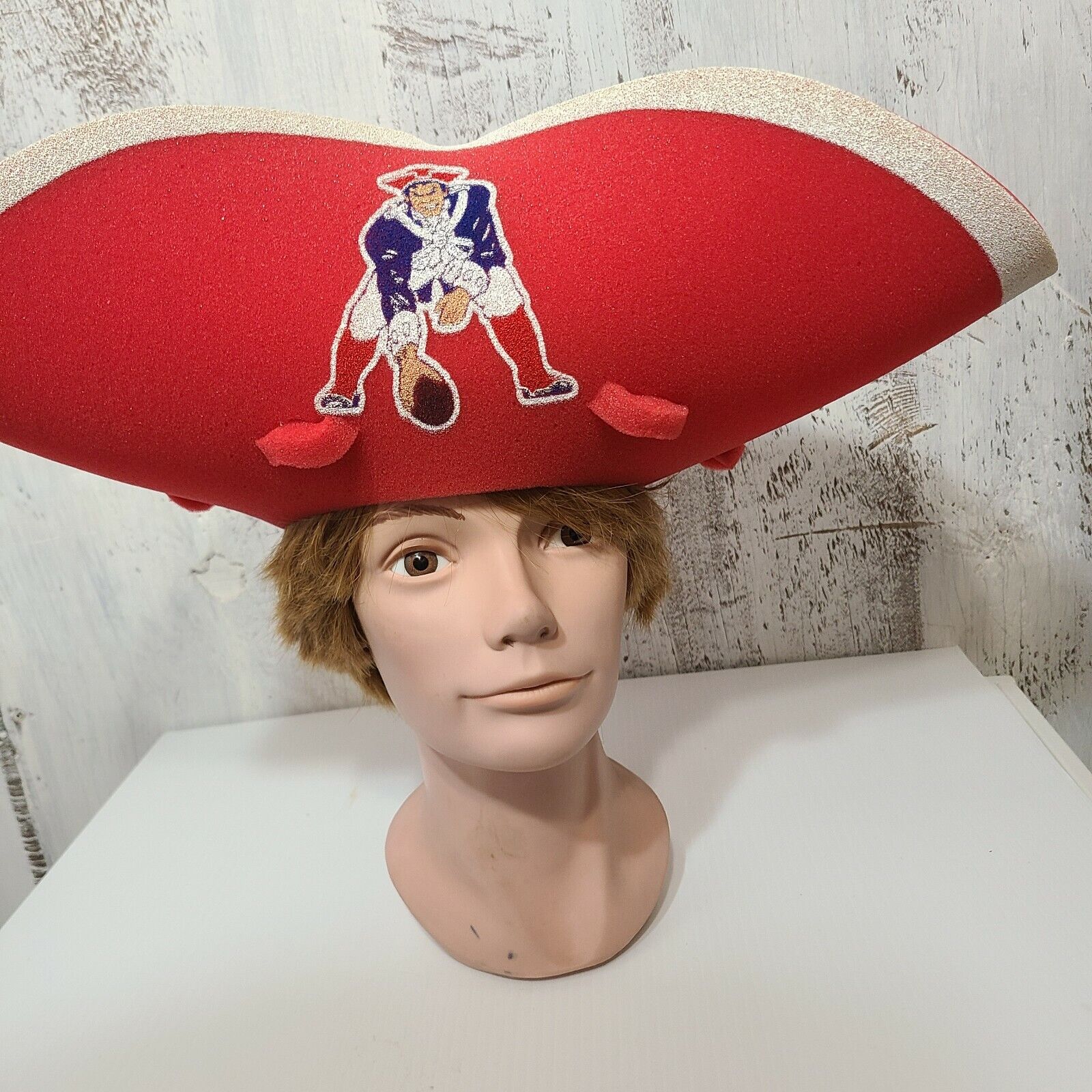The image captures a close-up photograph of a female mannequin head and neck, featuring pale skin, brown eyes, and short light brown hair with matching brown eyebrows. The mannequin faces directly toward the camera, placed on a white, distressed wooden surface. The background is a faux-grainy wood texture painted in white with brown accents, contributing to a rustic aesthetic. Adorning the mannequin's head is a unique, old-fashioned red hat with a white trim, reminiscent of a Napoleon Bonaparte-style or an 18th-century sailor's cap. This hat depicts an illustration of a character dressed as a red, white, and blue pirate from a bygone era, bending over to hold a football. This pirate-like figure wears red socks, white pants, a blue top, and a white scarf, styling that evokes the fashion of the 1700s.